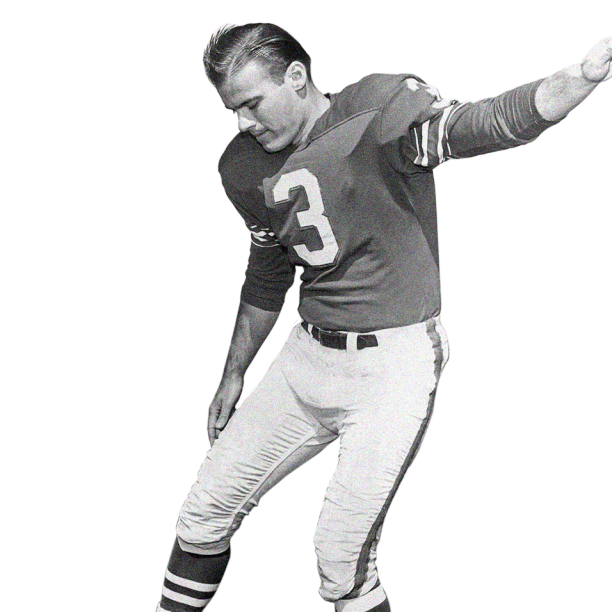This is a detailed black and white photograph of a mid-20th century American football player, likely from the 1950s or 60s. The player, a white male with a clean-cut, boyish haircut, stands as the central focus against a white background, dressed in professional football attire. He wears a dark-colored jersey adorned with the number three and white lettering, accompanied by shoulder guards and white pants featuring a dark line along the sides. His outfit is completed with a black belt and high black socks with two white stripes.

The player is looking down contemplatively at his right foot, which is slightly extended as if he is preparing to kick or nudge something out of the frame. His right arm reaches towards his right knee, while his left arm is raised upward, extending beyond the edge of the photo. His posture, with one leg firmly planted and the other slightly elevated, and his focused gaze contribute to the impression that he is in the middle of a kicking motion. The image is cropped so that parts of his hands and feet are not visible, but his expression and the positioning of his limbs suggest a moment of concentration and athletic readiness.